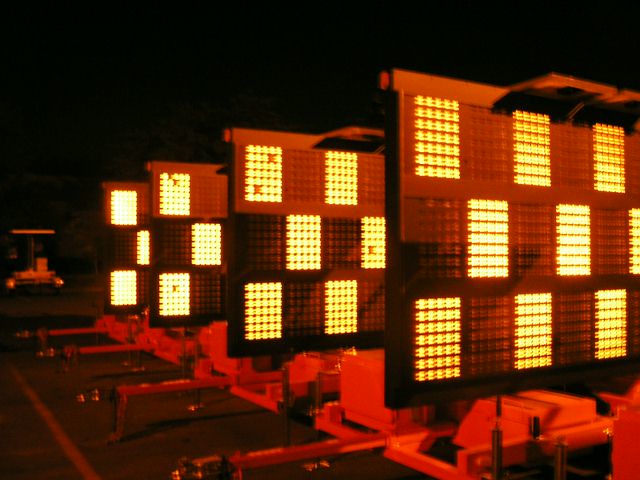The image depicts four traffic display panels mounted on mechanical platforms, illuminated under an orange-red light in an otherwise dark setting. Each panel features a distinct checkerboard pattern made up of small light grids with alternating illuminated and unlit sections, arranged in a 5x6 grid format. The top rows feature a pattern of lit-white and unlit segments, while the bottom row reverses this sequence. The background is predominantly black, making it difficult to ascertain whether the scene is indoor or outdoor. However, a white vehicle or trailer is visible in the background, suggesting an outdoor location. The panels seem poised for programming to display various characters or numbers. The overall scene showcases a mysterious and mechanically complex arrangement, possibly hinting at a large-scale application or installation.